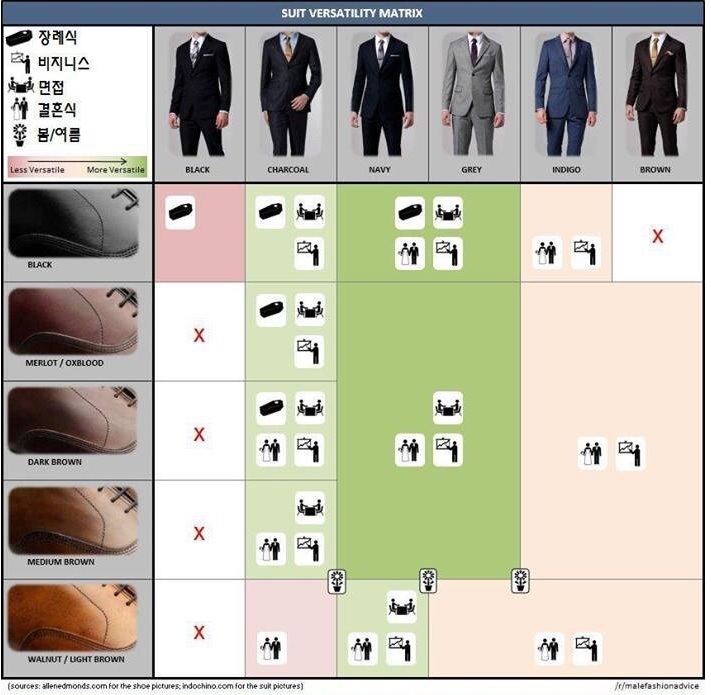In this photograph, there is a detailed "Suit Versatility Matrix" designed as a guide to help piece together the perfect men's suit and shoe combinations. The top left corner includes a key with several characters indicating gender and what looks like Chinese or Korean symbols. A gradient graphic spans horizontally from light red to green, labeled "less versatile" to "more versatile" from left to right. The matrix itself lists various suit colors along the top row: black, charcoal, navy, gray, indigo, and brown. Below each suit color, corresponding shoe colors are listed in a vertical column: black, merlot/oxblood, dark brown, medium brown, and walnut/light brown. The table appears to indicate the versatility of each suit and shoe combination, with specific colors and symbols, including Xs, illustrating appropriate matches for different situations. Further details, such as more human symbols, are located at the bottom right-hand corner, adding to the comprehensive nature of this visual guide.